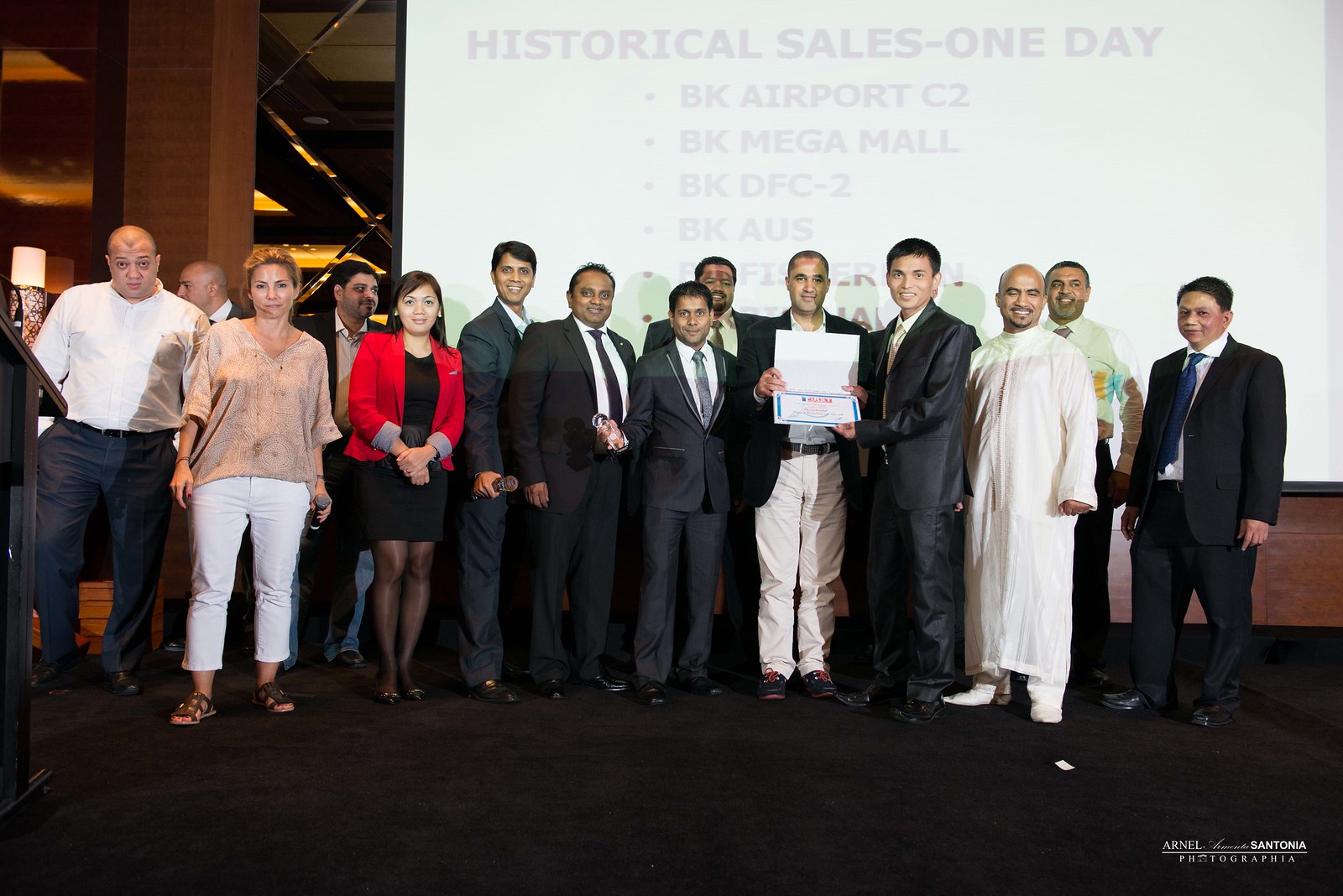The image is a color photograph capturing a formal event featuring a large group of people, predominantly men, with two women prominently positioned in the front row. All are smartly dressed, ranging from black business suits to traditional attire, suggesting a diverse group that includes Caucasian, Chinese, and Indian individuals. The setting appears to be a business conference or award ceremony, as indicated by the central figure holding what seems to be a certificate or award. Behind the group is a white screen with black text that reads "Historical Sales - One Day," followed by a list of bullet points: BK Airport C2, BK Megamall, BK DFC2, and BK AUS. The background also includes faint images and mirrors, indicating the setting might be a hotel or conference hall, with "Arnold Santonia Photographia" inscribed at the bottom of the image.